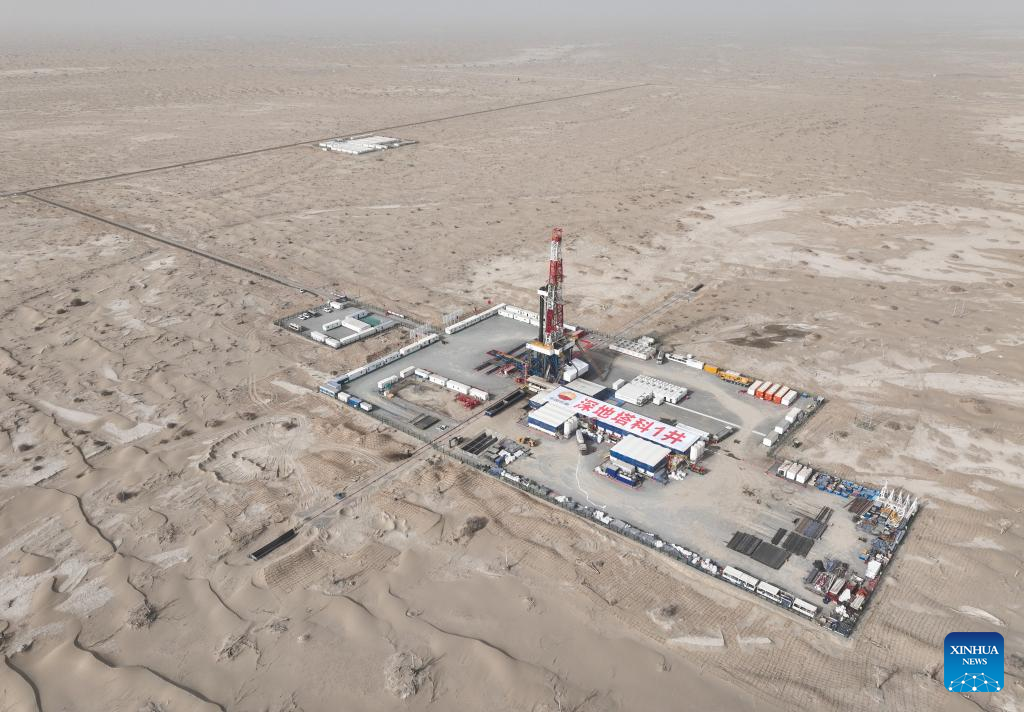This aerial photograph showcases a sprawling compound situated in a light-colored, arid desert landscape that stretches for miles in all directions. At the center of the image, surrounded by sand with no vegetation in sight, there is a rectangular concrete pad featuring various buildings and infrastructure elements. Prominent among these is a tall, red and white crane, likely associated with oil drilling operations, suggestive of an oil welling platform akin to those used on ocean oil rigs. The compound's structures include worker's buildings with Chinese lettering on the roof, indicating that this facility is either in China or operated by a Chinese company. There are several storage containers dispersed around and inside the perimeter of this rectangular island-like compound. Also visible are various vehicles, possibly rows of cars or cargo containers in the distance, signifying significant logistical activity. The bottom right corner of the image prominently displays the logo of Xinhua News, a Chinese news agency. Despite the general grey tone of the photograph, the red elements on the crane and the lettering on the buildings stand out, adding slight coloration to the scene.